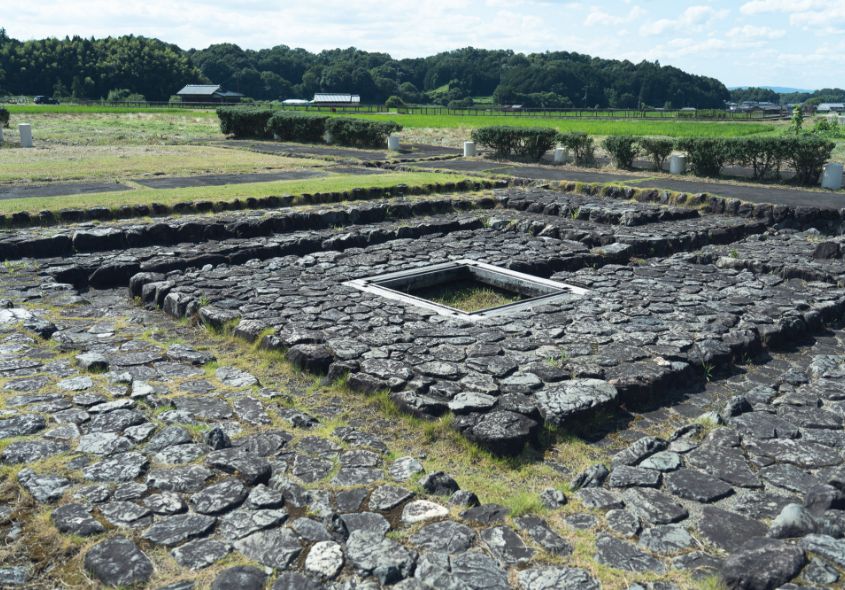The image depicts the ruin of an ancient stone castle situated in a lush, green countryside. The central focus is the stone foundation, characterized by rectangular and square shapes, delineated by clusters of grey stones. In the middle of the ruins is an open square bordered by what appears to be metal, allowing the grass underneath to peek through. Surrounding the ruin is the outline of an old moat, now dry and possibly filled with grass. Beyond the stone remnants, the landscape expands into verdant fields, with green hedges and a forest in the far distance. Farmhouses or barns dot the horizon, under a wide, blue sky with scattered white clouds. The overall scene exudes tranquility and the timeless beauty of rural landscapes, captured in the serene daylight.